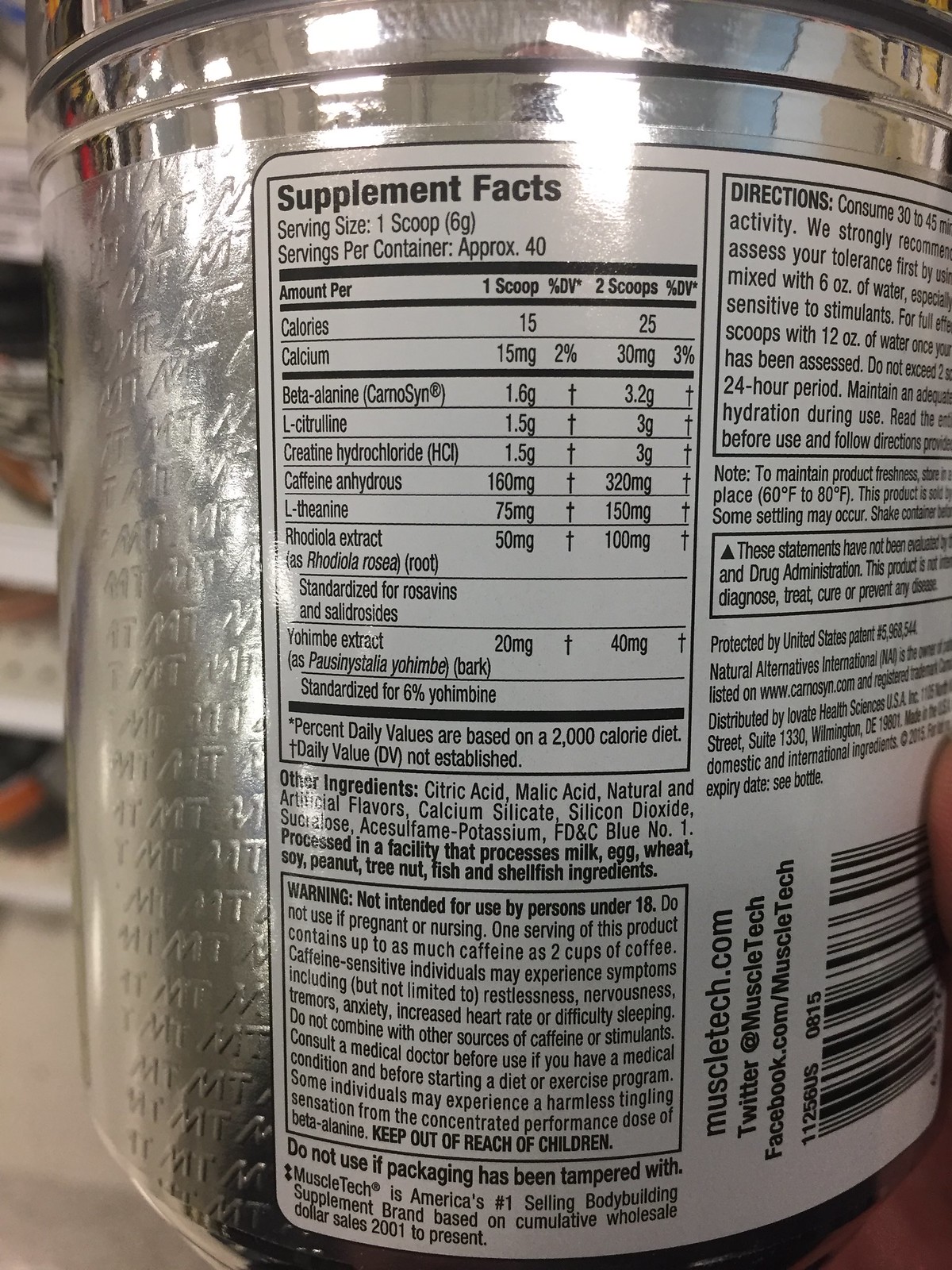A detailed close-up image of a gleaming silver container captures the viewer’s attention with its shiny surface reflecting ambient light. The container boasts a label at the back, prominently titled "Supplement Facts." According to the label, each serving size of the product is one scoop, with around 40 servings per container. It provides nutritional details including calories, calcium, creatine, and caffeine, with daily value percentages based on a 2,000 calorie diet. Additional ingredients are listed, with citric acid being the first. A warning specifies that the product is not intended for individuals under 18. Directions for use are clearly stated, and the container also features a SKU for scanning, along with details of the manufacturing company and their email address for contact.